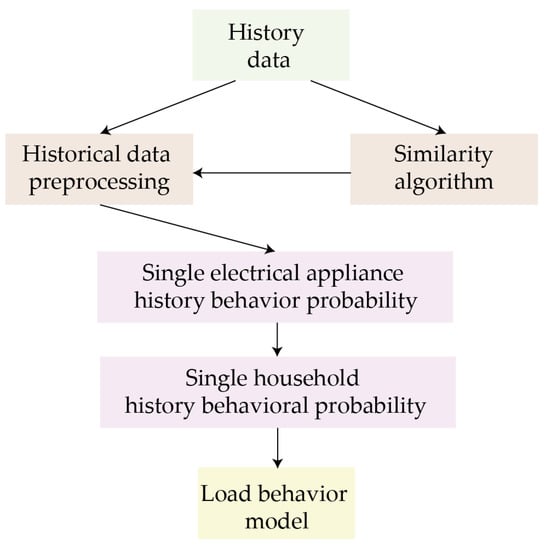The image is a detailed flowchart consisting of six rectangles with specific steps and connections. At the top center is a pastel green rectangle labeled "History Data." From this, two arrows emerge, one pointing to the bottom left and the other to the bottom right. The bottom left rectangle, in beige, is labeled "Historical Data Pre-Processing," while the bottom right beige rectangle reads "Similarity Algorithm." An arrow from the "Similarity Algorithm" rectangle loops back to "Historical Data Pre-Processing," indicating interaction between these two steps.

Below the "Historical Data Pre-Processing" rectangle, an arrow points down to a soft pink rectangle labeled "Single Electrical Appliance History Behavior Probability." Another arrow extends downward from this to another soft pink rectangle labeled "Single Household History Behavioral Probability." Finally, a small black arrow leads from this rectangle to a pastel yellow rectangle at the bottom, which is labeled "Load Behavior Model." 

This detailed diagram visually represents the progression and interaction of various data processing stages, from historical data to the final load behavior model.